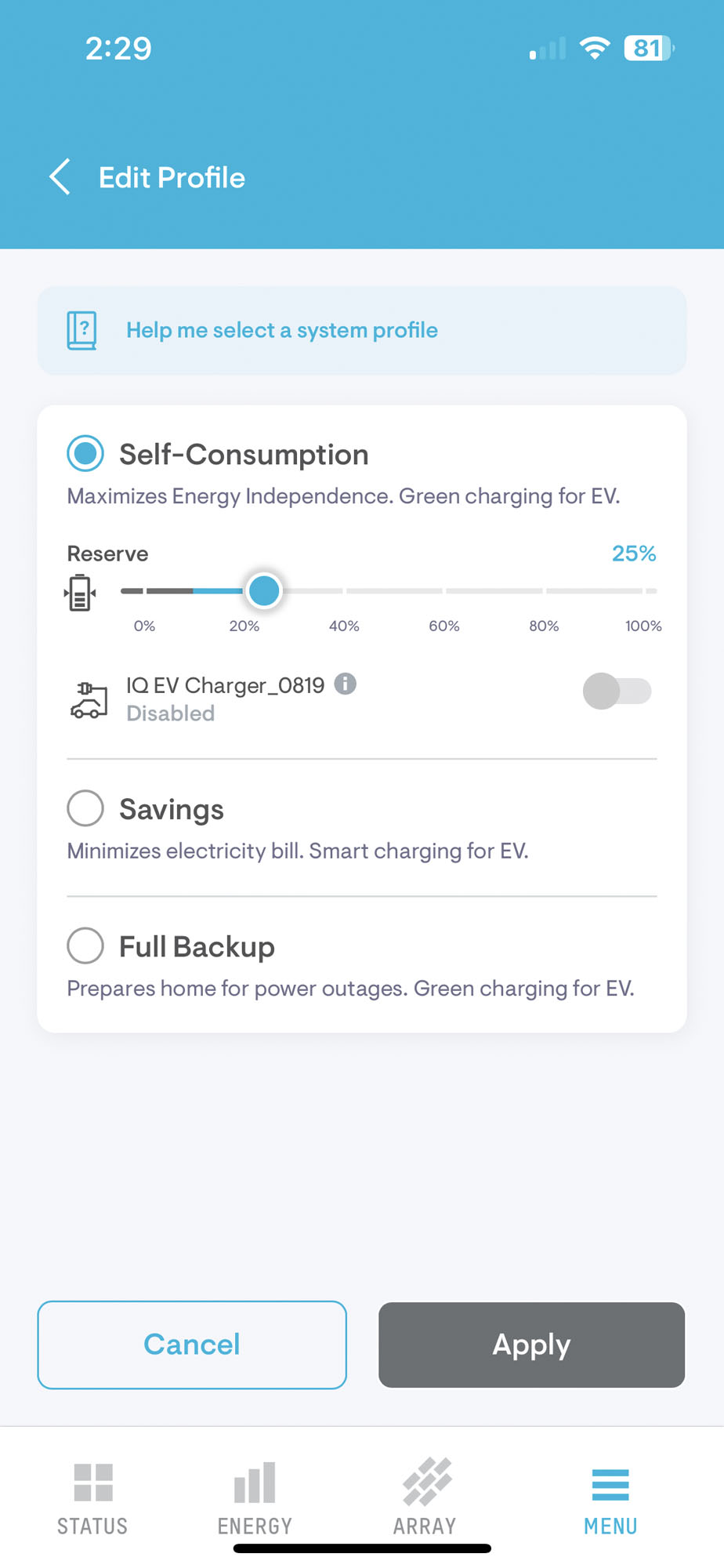The screenshot depicts a smartphone interface with a user-friendly energy management system. At the top, a baby blue banner displays the time, 2:29, alongside indicators for a strong Wi-Fi signal and an 81% battery level. Adjacent to these indicators are a left-facing arrow icon and an "Edit Profile" option.

Beneath this header, the interface transitions into a green section with baby blue text, prominently featuring a book icon with a question mark on its cover and the message, "Help me select the system profile."

Continuing downwards, a white box houses a blue button, matching the consistent blue theme, labeled "Self-Consumption: maximizes energy independence, green charging for EV."

Further below, a graph-like element illustrates a "Reserve" setting, ranging from 0% to 100%, with the current level set at 25%. 

An option named "IQ EV Charger_0819" appears next, indicated as disabled. Adjacent buttons for "Savings" (unselected) and "Full Backup" (also unselected) provide additional functionalities. "Savings" aims to "maximize electricity bill, smart charging for EV," whereas "Full Backup" is designed to "prepare home for power outages, green charging for EV."

Lastly, two buttons at the bottom offer actions: "Cancel" and "Apply." The bottom navigation bar includes tabs labeled "Status," "Energy," "Array," and "Menu," with the "Menu" tab currently active.